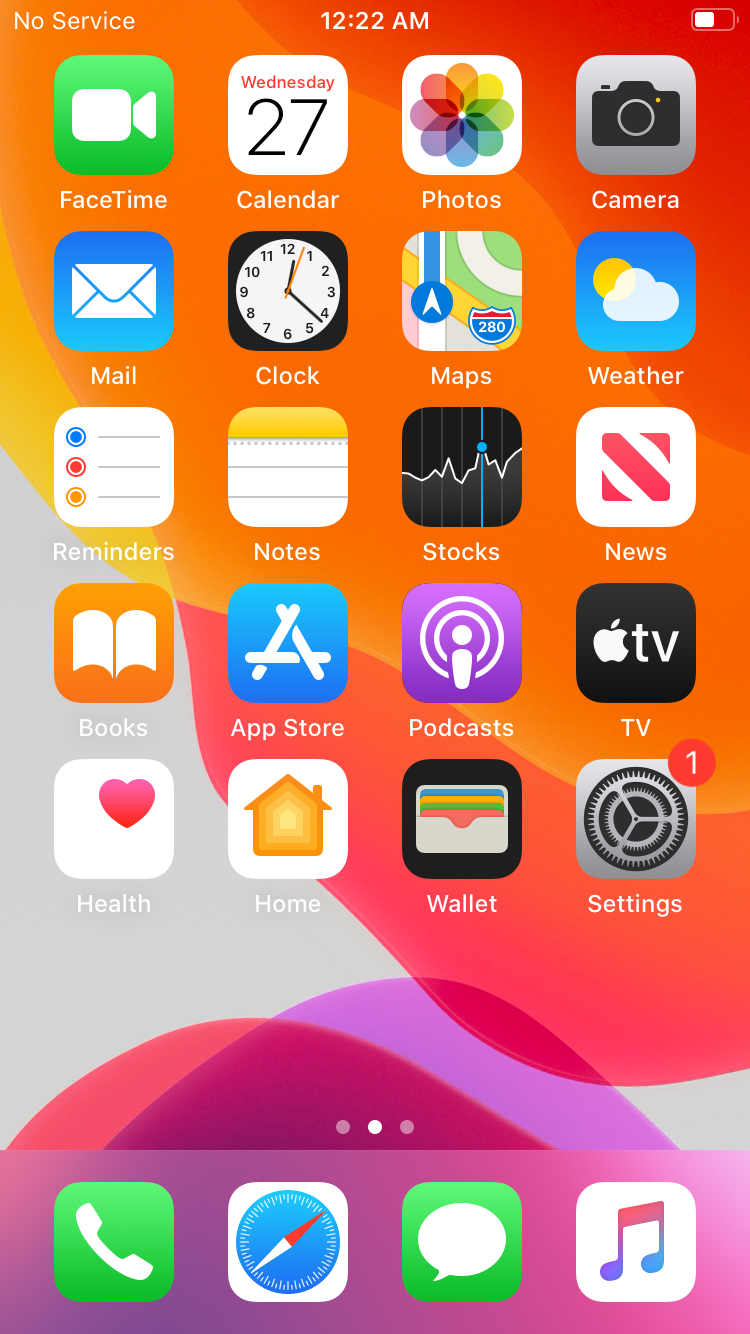This image showcases an Apple iPhone screen with a clear display at 12:22 AM. The device is not connected to any network, as indicated by the "No Service" message to the left of the time, and the battery icon on the right shows it is half full. The vibrant background features a dynamic swirl pattern in shades of orange, magenta, purple, pink, and white.

The home screen is organized with a variety of app icons, reflecting a typical arrangement of an iPhone's default applications. From top to bottom, the first line includes the FaceTime, Calendar, Photos, and Camera apps. The second line features the Mail, Clock, Maps, and Weather apps, while the third line comprises Reminders, Notes, Stocks, and News apps.

Following this, the Books, App Store, Podcasts, and TV apps occupy the next row, with another line below housing the Health, Home, Wallet, and Settings apps, the latter of which has a notification badge showing '1'. Below these apps, dots indicate additional home screens for navigation.

At the bottom dock, distinct app icons include the Phone app for calls, Safari for web browsing, Messages for chatting, and Music for audio playback, all providing quick and essential access for the user.